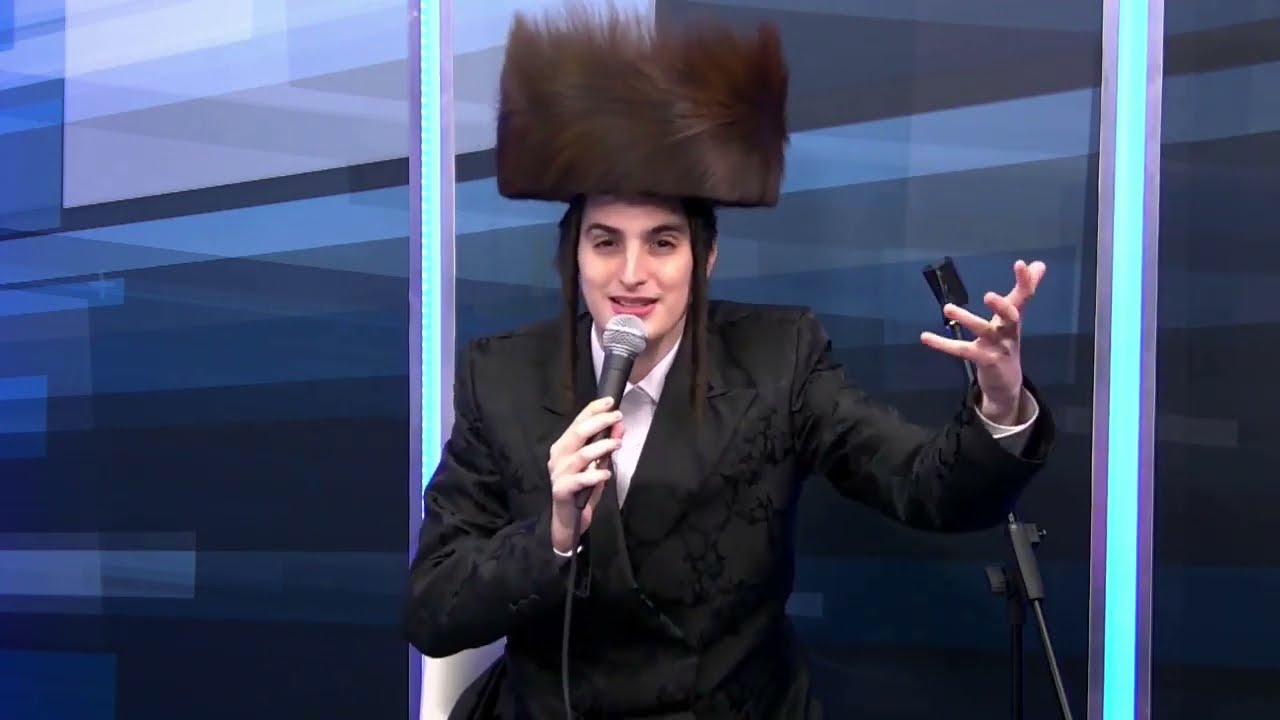In the image, a young man, centered and seemingly in mid-performance, stands against a vividly colored background featuring an array of purples, aqua light blues, and various shades of blue, interspersed with vertical green lines bordered by purple stripes. He dons a stylish black suit jacket adorned with intricate, darker black floral patterns, over a pristine white collared shirt. His fair, peach-toned complexion contrasts sharply with his large, round, furry brown hat, which fits snugly atop his head and features two braided straps hanging down the sides of his face. In his right hand, he holds a microphone close to his lips, his arm bent at the elbow. His left arm is also raised, with his palm open, gesturing expressively in front of a microphone stand positioned slightly behind him. The overall scene suggests he is delivering a speech or perhaps performing, with the background’s dynamic artwork adding a sense of energy to the moment.